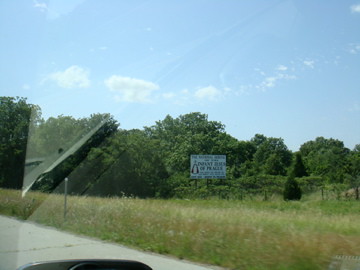Outdoor photo taken from inside a car, capturing the dashboard on the lower left and a slight windshield reflection, against a backdrop of a blue sky with a few clouds. Below the sky, there's a horizon of lush trees, some close to the car. A distant white sign with illegible text nestles under one of the trees, suggesting a billboard or significant larger sign, possibly on private property. To the right of the sign is a pasture housing a single horse. The road is visible in the foreground, with a patch of green grass and some reddish plants. A sidewalk is discernable in the lower left, enhancing the sense of driving through a rural or Midwestern landscape.